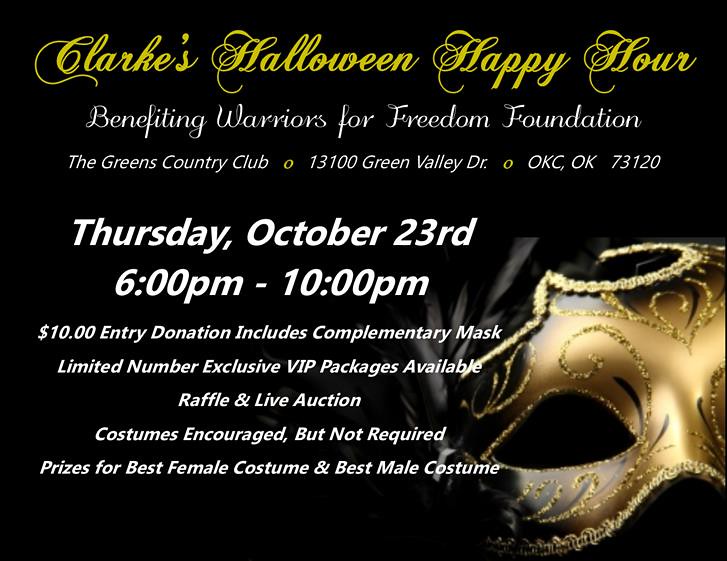This advertisement for Clark's Halloween Happy Hour features a striking black background with text in white and yellow. At the top, "Clark's Halloween Happy Hour" is elegantly written in cursive white font. Below, in white lettering, details about the event are presented: Benefiting Warriors for Freedom Foundation, held at The Greens Country Club, 13100 Green Valley Drive, Oklahoma City, OK 73120. The event is scheduled for Thursday, October 23rd from 6 p.m. to 10 p.m. with a $10 entry donation that includes a complimentary masquerade mask. Exclusive VIP packages are available in limited numbers. Additional event highlights include a raffle and live auction, with costumes encouraged but not required. Prizes will be awarded for the best female and male costumes. To the lower right, the advertisement features a cropped image of a decorative masquerade ball mask.